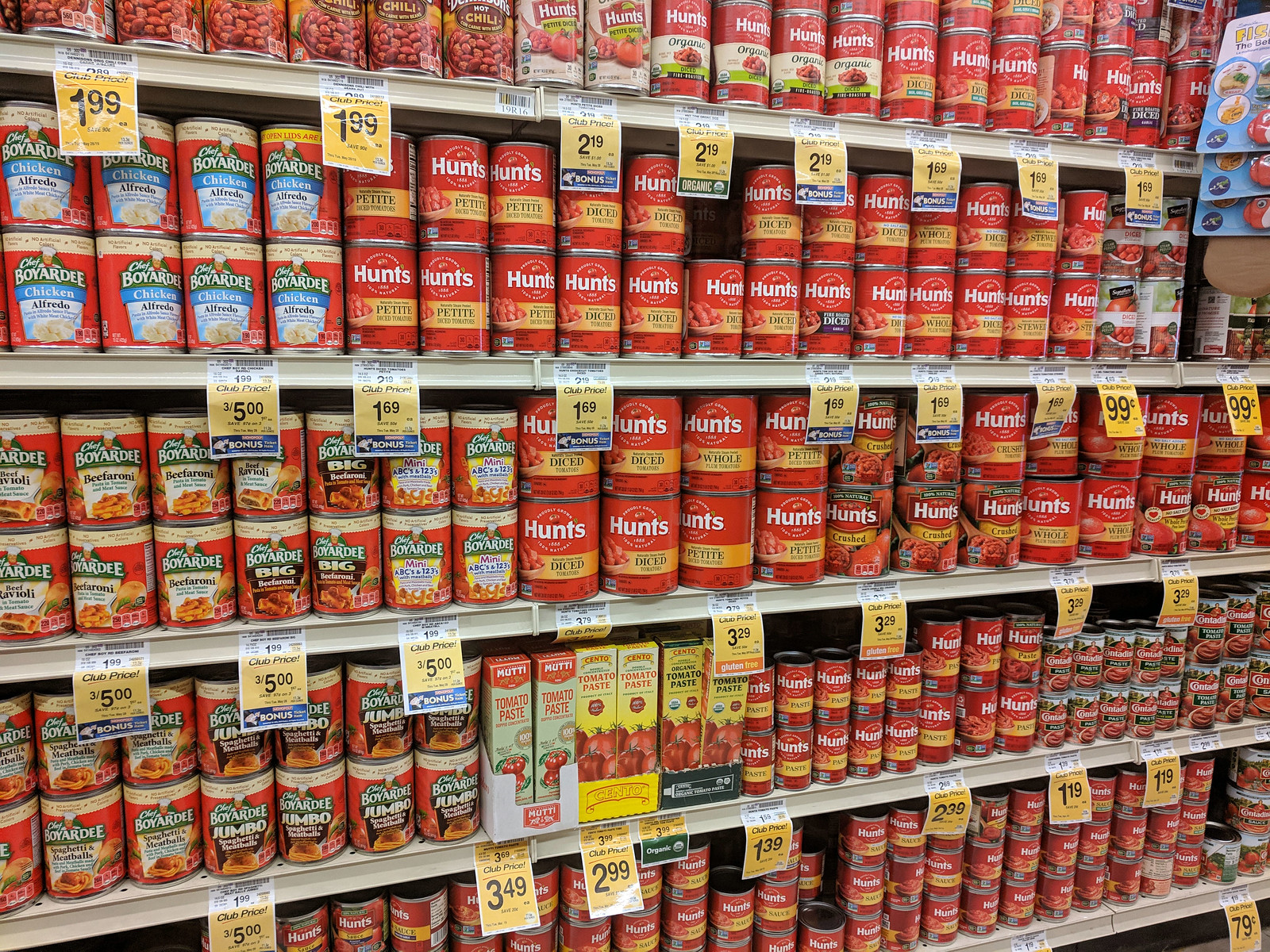The image captures a well-organized display of five grocery store shelves stocked with various canned goods. 

- **Top Shelf:** Lined neatly with cans of hot chili beans, multiple varieties of Hunt's tomatoes including standard and organic options, and more Hunt's tomato products.
- **Second Shelf:** Displays an assortment of Chef Boyardee Chicken Alfredo cans, Hunt's Petite and Diced Tomatoes, and another brand of Diced Tomatoes on the far right.
- **Third Shelf:** Features cans of Chef Boyardee Beef Ravioli, Chef Boyardee Mini ABCs and 1-2-3s, alongside more Hunt's Diced, Crushed, and Whole Tomatoes.
- **Fourth Shelf:** Contains Chef Boyardee Spaghetti and Meatball cans, Chef Boyardee Jumbo Spaghetti and Meatballs, boxes of Muir Glen Tomato Paste, Cento Tomato Paste, and various sizes of Hunt's and Contadina Tomato Paste.
- **Bottom Shelf:** Offers additional Hunt's Tomato products including Tomato Sauce and Contadina Tomato Sauce.

Price tags are affixed to the edge of each shelf, providing clear pricing information for shoppers.